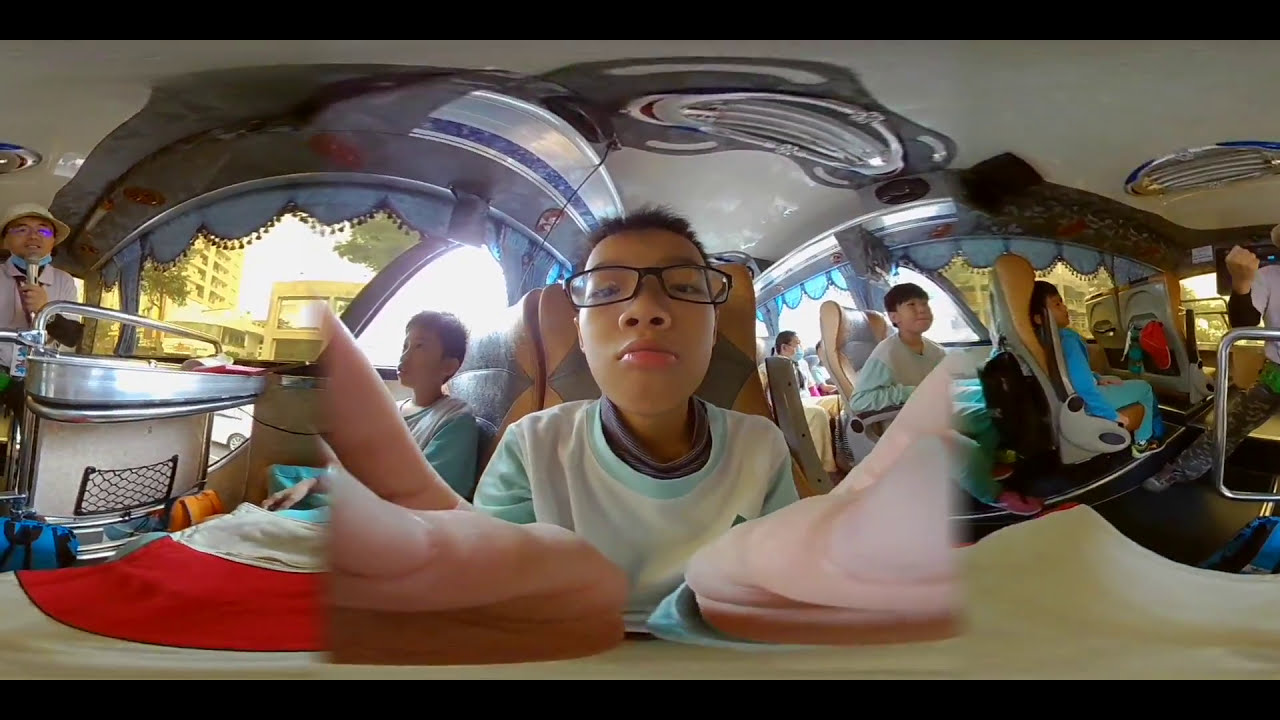The image features a young Asian boy, likely in elementary school, sitting at the center of a bus with a city backdrop visible through the windows. He is wearing a light blue sweater with blue trim and black, rectangular glasses. The young boy appears to be fiddling with something in front of him, possibly holding the camera, creating a focus on his face and hands. Surrounding him, several passengers are seated on white cushioned seats. On the left side of the image, an Asian man wearing a beige bucket hat and a blue face mask on his chin is holding a silver microphone, presumably acting as a tour guide. The bus has a spacious interior with a white ceiling and blue scalloped fringes around the windows. Other passengers, including women and children, are attentively listening to the tour guide.